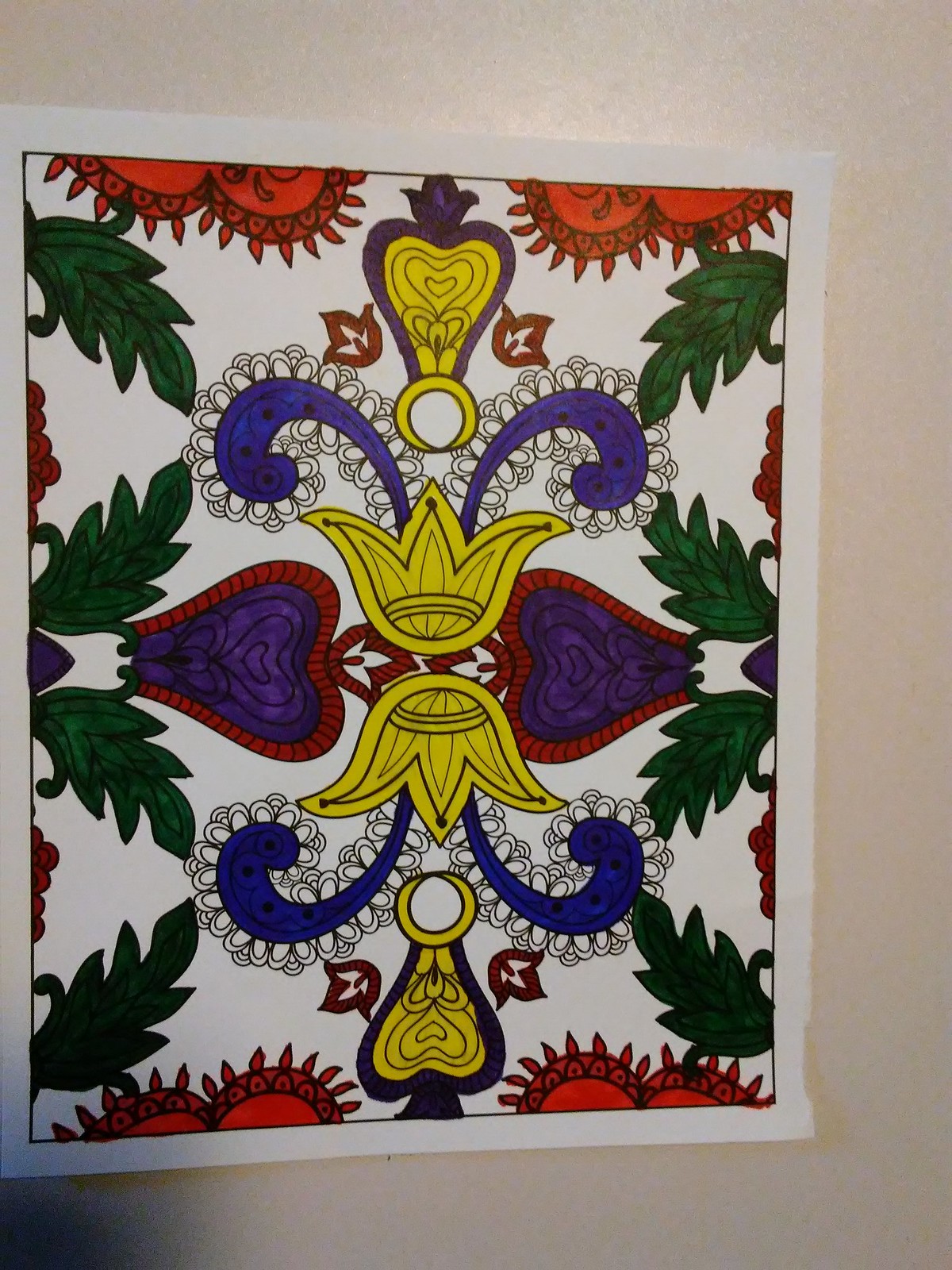This photo showcases a colorful, detailed artwork that closely resembles a page from an adult coloring book or the back of a playing card. The intricate design is characterized by interlocking heart-shaped motifs, flowers, curlicues, and leaves, all outlined in black and filled in with vibrant markers. Dominating the center of the artwork are two gold crowns, reminiscent of a fleur-de-lis, with one facing upward and the other downward. Flanking the crowns are heart-shaped elements with purple interiors and gray and red exteriors, mirrored above and below like onions. The pattern continues with a border of red flaming hearts and clusters of green leaves—four on each side—along with blue paisleys that curl around the crowns. These paisleys are predominantly purple and adorned with white flowers, completing the rich, colorful tapestry that could either be placed on a white table or mounted on a wall.